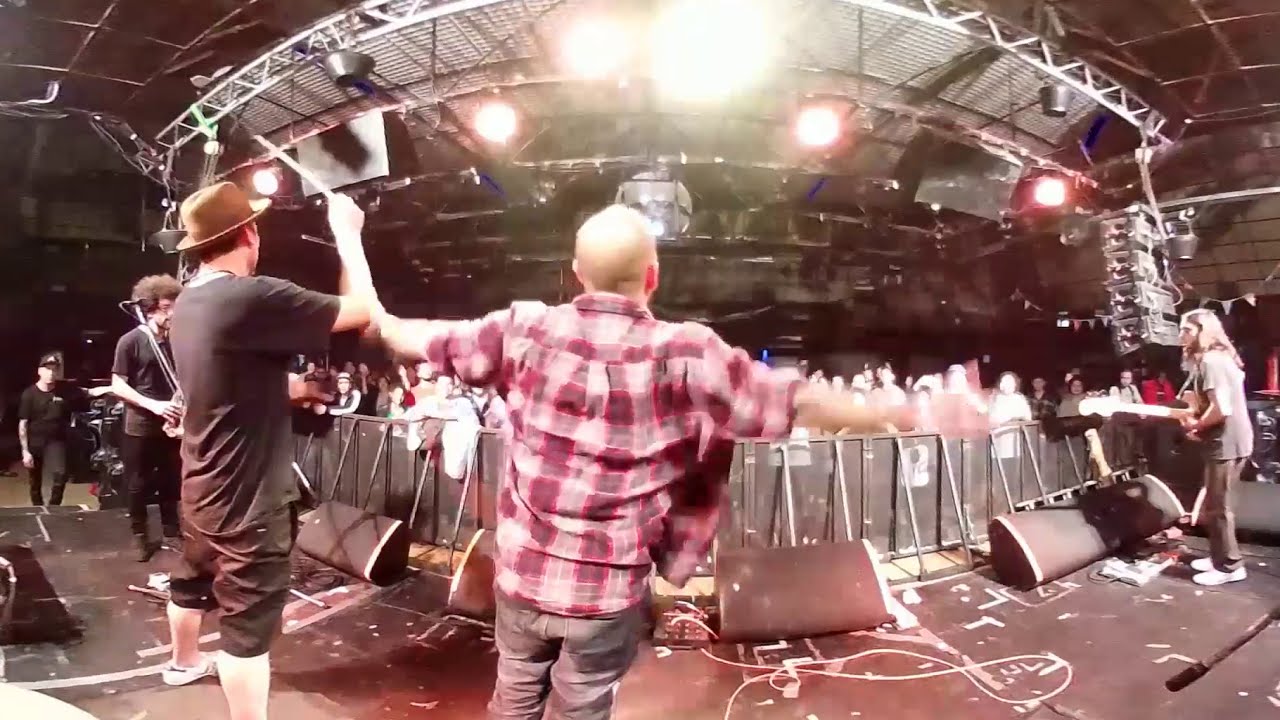In an indoor concert setting, the image captures a vibrant scene from a curved perspective. At the forefront of the picture, a bald man in a red plaid shirt and gray pants is energetically waving his arms, illuminated by overhead stage lighting. To his right, a person with long hair, wearing a gray short-sleeved shirt, pants, and white shoes, stands out. On the left side, another person in a dark t-shirt and shorts, along with a brown hat, holds up a drumstick, seemingly engaging with the crowd. The stage, surrounded by barriers, is equipped with sound equipment and various speakers, with people both seated and standing around it. The floor shows signs of a lively event, littered with trash and a white cord. The scene is framed by a backdrop of lights, some brighter than others, encapsulating the buzz and energy of the concert.